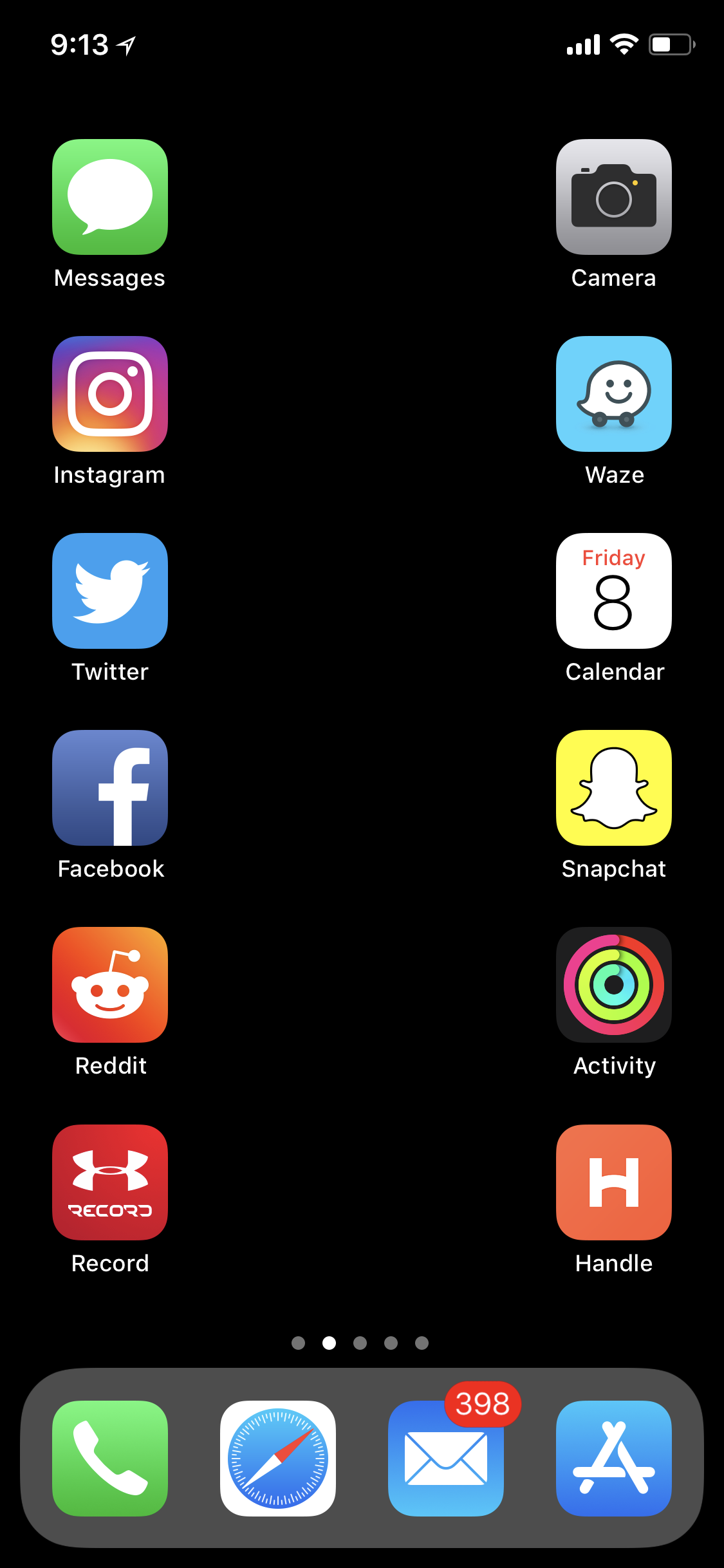The image displays the home screen of an Android smartphone, set against a black background. The top left corner of the screen shows the time, "9:13," followed by an icon indicating that the location settings are enabled. Below this, the screen is organized into a grid of application icons with corresponding labels:

- **Messages**: Icon followed by the label "Messages".
- **Instagram**: Icon followed by the label "Instagram".
- **Twitter**: Icon followed by the label "Twitter".
- **Facebook**: Icon followed by the label "Facebook".
- **Reddit**: Icon followed by the label "Reddit".
- **Record**: Icon followed by the label "Record".

On the right-hand side, at the very top, the status indicators show full signal bars and active Wi-Fi, with the battery icon indicating a half-full battery. Below this, an additional list of application icons and labels appears:

- **Camera**: Icon followed by the label “Camera”.
- **Waze**: Icon followed by the label "Waze".
- **Calendar**: The display shows the date "Friday the 8th" with the "Calendar" label beneath.
- **Snapchat**: Icon followed by the label “Snapchat”.
- **Activity**: Icon followed by the label "Activity".
- **Handle**: Icon followed by the label "Handle".

At the bottom of the screen, four frequently used apps are docked:

- **Phone**: Icon for making calls.
- **Weather**: An icon likely representing a weather app.
- **Email**: Icon indicating 398 unread emails.
- **Unknown App**: An icon shaped like an 'A', the purpose of which is unclear.

Overall, the screen is neatly organized, providing easy access to various social media, utility, and functional applications.